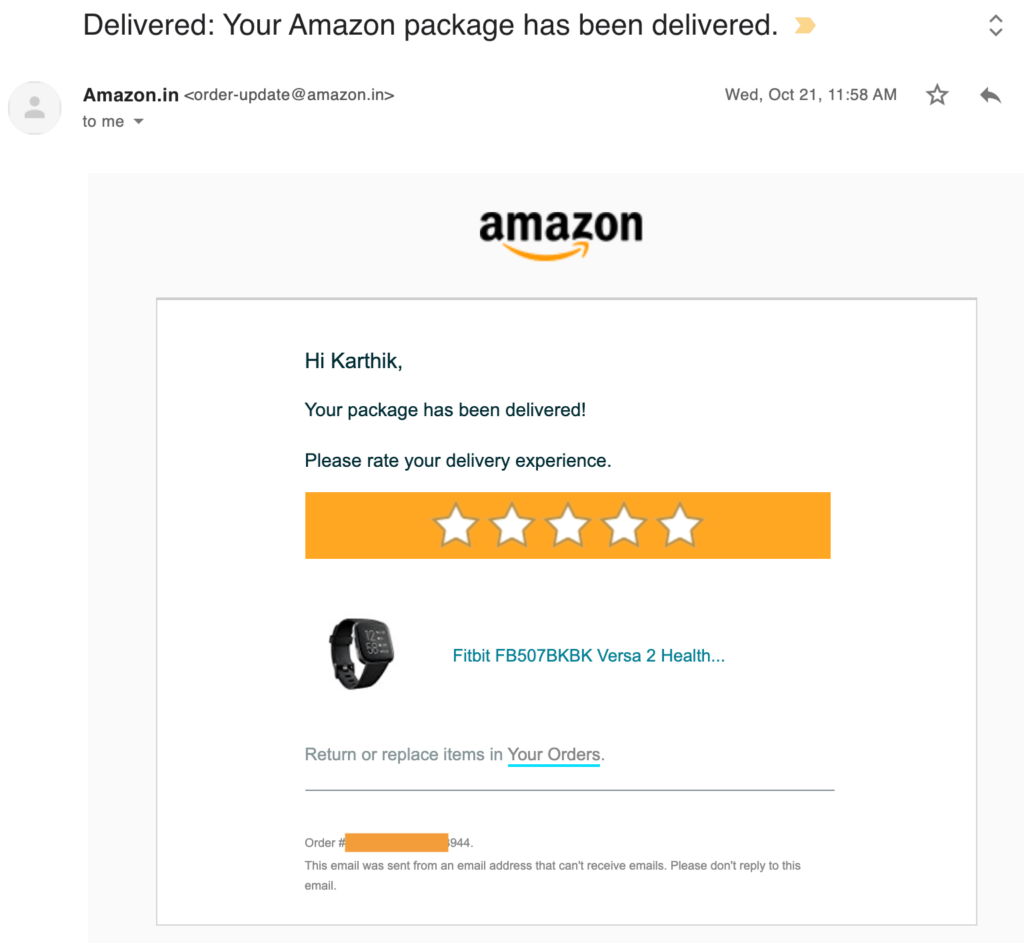The image is a screenshot from a smartphone displaying an Amazon delivery confirmation message. At the top, there's a notification stating, "Delivered: Your Amazon package has been delivered," accompanied by a yellow arrow pointing to the right. Below this, the text "amazon.in" is visible, indicating the source of the message. The recipient’s name is noted as "To: Me."

To the right of this, the date "Wednesday, October 21" and the time "11:58 AM" are displayed, followed by a star and a return arrow icon. Beneath this, the Amazon logo appears within a faint gray square.

In the main body of the message, the text reads, "Hi Karthik, your package has been delivered. Please rate your delivery experience." Below this, there is a clickable rectangle containing five white stars for rating the delivery.

An image of the delivered item is shown next: a black Fitbit with the partial product name "Fitbit Versa 2 Health…" Below the image, there's an option to "Return or Replace Items in Your Orders" with a blue teal underline indicating a clickable link.

The message concludes with some small print at the bottom and a small yellow rectangle, possibly containing additional action buttons or information.